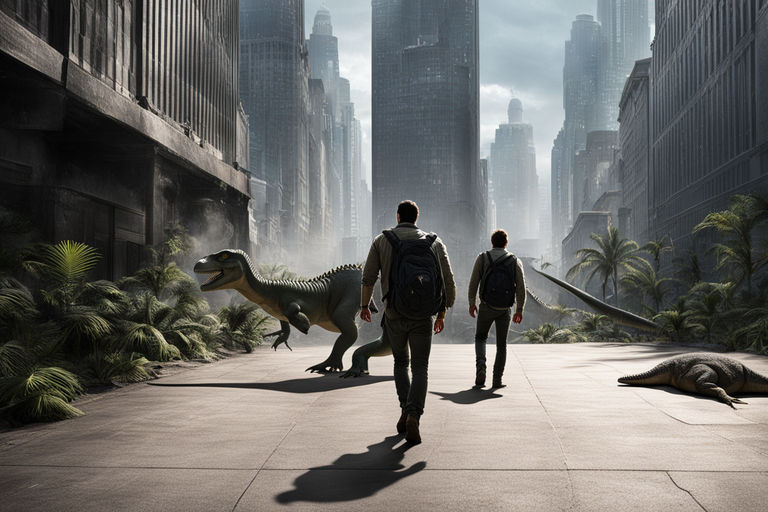In this AI-generated animated image, we observe an apocalyptic cityscape engulfed in fog, with looming skyscrapers fading into a hazy backdrop. Central to the scene are two men, dressed in long-sleeved jackets and pants, walking forward with backpacks. Their shadows stretch behind them as they navigate the concrete floor. Directly ahead, a carnivorous dinosaur, likely a velociraptor, confronts them, yet they appear undaunted. To the side, a large dinosaur, potentially resembling a crocodile, lies flat on the ground. The city is strangely overgrown with tree-like bushes and ferns sprouting from the concrete, lending an eerie blend of natural and urban decay. This surreal juxtaposition of futuristic ruin and prehistoric life creates a poignant visual narrative possibly commenting on the unchecked consequences of advanced technologies like global warming and DNA manipulation.